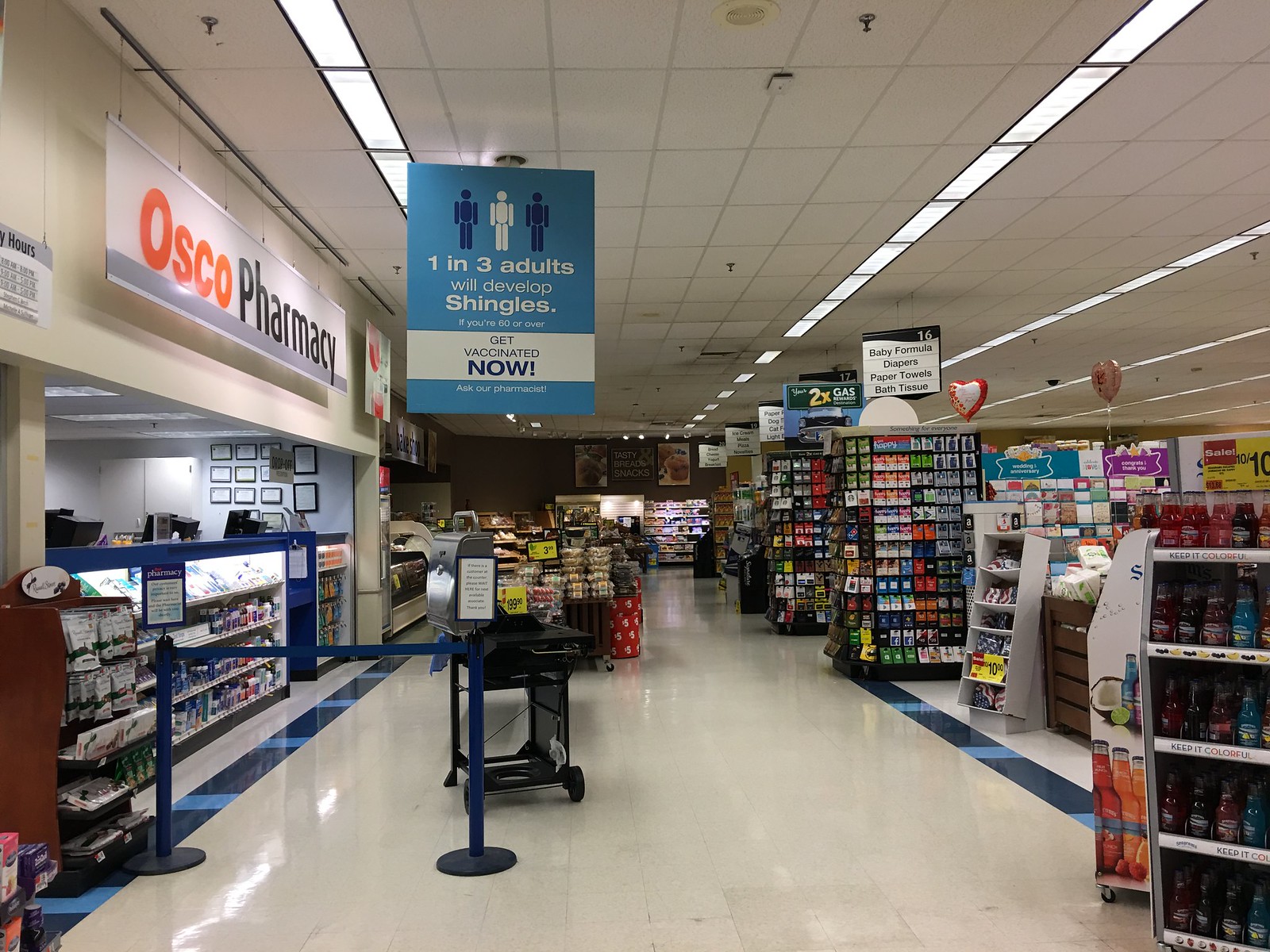This photograph was taken inside an Osco pharmacy located within a grocery store. On the left side of the image, a prominent sign displays "Osco Pharmacy" in red and black lettering. In front of the pharmacy counter, shelves are stocked with various items available for purchase, while a blue rope guides customers in line. Hanging from the ceiling is a blue banner featuring line drawings of three individuals—two in blue and one in white—alongside a health advisory that reads, "One in three adults will develop shingles. If you're 60 or over, get vaccinated now. Ask our pharmacist."

The background teems with various goods, suggesting a comprehensive grocery store environment. Several tables laden with baked goods are prominently visible, reinforcing the grocery store setting. On the right side of the image, there are racks filled with beverages and an aisle dedicated to greeting cards. Nearby, multiple racks showcase a variety of gift cards. Additionally, two heart-shaped helium balloons float to the right, adding a festive touch. A sign indicating "Aisle 16" lists items such as baby formula, diapers, paper towels, and bath tissue. In the far background, additional signs are partially visible, and the ceiling is lined with fluorescent lights that brightly illuminate the space.